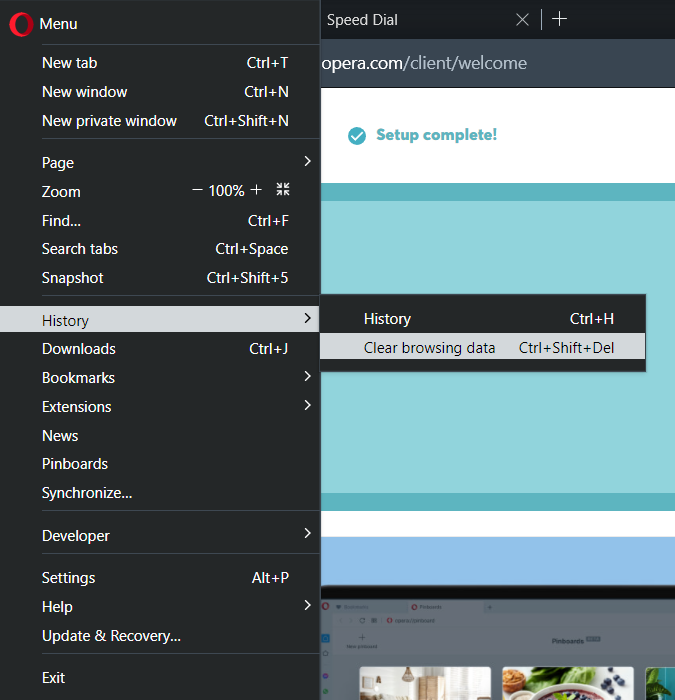This is a screenshot of the menu page for the Opera web browser. The interface features a black background on the left side of the menu, with contrasting gray, white, and blue areas on the right. 

In the top left corner, the iconic Opera logo—a red "O"—is prominently displayed, followed by the word "Menu." 

The menu options are listed vertically in a clear and organized manner along the left side of the screen. These options include:

- New Tab
- New Window
- New Private Window
- Page
- Zoom
- Find
- Search Tabs
- Snapshot
- History
- Downloads
- Bookmarks
- Extensions
- News
- Pinboards
- Synchronize
- Developer
- Settings
- Help
- Update and Recovery
- Exit

The "History" option is highlighted, indicating it is currently selected. To the right of the main menu, there is a section featuring a right-pointing arrow, and immediately next to it are the options "History" and "Clear Browsing Data." This layout suggests an intuitive design focused on user accessibility and functionality.